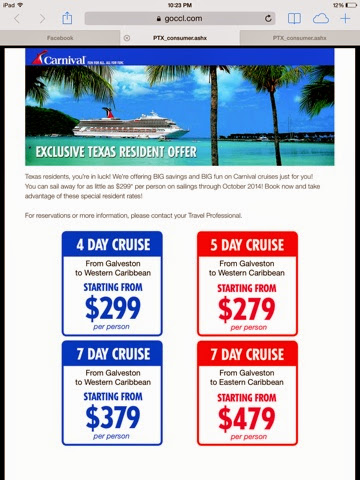An image, cropped from a mobile screenshot, features a gray header section at the top of the phone display, which includes the time, address bar, and icons such as the battery symbol in the top right corner. The main section, surrounded by a black border on the left, right, and upper sides but cut off at the bottom, rests against a white background. The header highlights three tabs labeled Facebook, PTX, and another PTX, with the center PTX tab selected. At the top of the main content area is an image of a Carnival cruise ship accompanied by the Carnival logo. Below the image reads "Exclusive Texas Resident Offer" in bold text, followed by a few lines of small gray text. Beneath this, the content is organized into four highlighted boxes displaying various cruise options and prices. On the left, two blue boxes list a "4-day cruise from $299" and a "7-day cruise from $379." On the right, two red boxes offer a "5-day cruise from $279 per person" and a "7-day cruise from $479 per person."